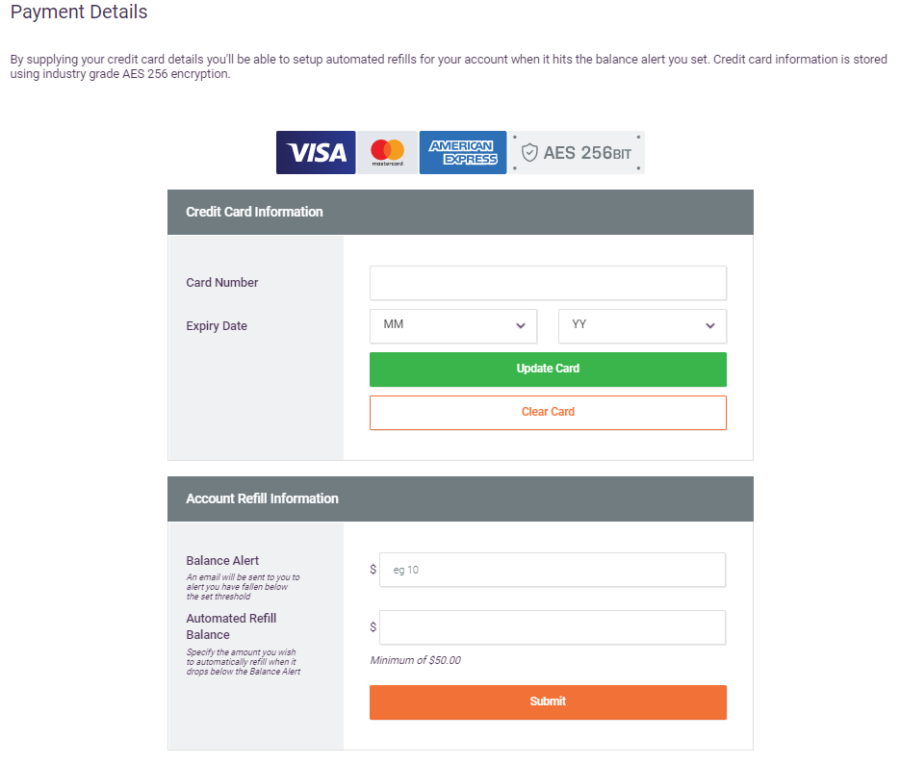### Caption:
This image is divided into multiple sections against a white background. In the upper left corner, the heading "Payment Details" is prominently displayed. The accompanying text explains that by providing your credit card details, you can enable automated refills for your account when it hits the user-defined balance alert. It ensures security by stating that credit card information is stored using industry-grade AES-256 encryption.

Centrally aligned in the next row are icons for Visa, MasterCard, and American Express, with a gray label to the right indicating "AES-256 bit". Below this, a dark gray stripe runs across, leading to a subsection on credit card information. This part of the image features a form with a left-aligned gray background that reads "Card Number" and "Expiry Date". Underneath, you can enter the card number in a rectangular field, and then select the expiry month (MM) and year (YY) from drop-down menus situated to the right.

Further below is a conspicuously large green button labeled "Update Card" in very tiny font, creating a sense of wasted space due to its disproportionate size. Adjacent to it, an orange-bordered button with small-font text states "Clear Card", also surrounded by a lot of unused space.

Following this, a large gray stripe labeled "Account Refill Information" introduces another form area. On the left, a column titled "Balance Alert" mentions that an email will be sent to notify you when your account balance falls below the set threshold. However, this text is hard to read due to its gray-on-gray italicized format. Directly below, the "Automated Refill Balance" description in italics and gray encourages users to specify the amount to automatically refill when the balance dips below the alert threshold. Here, users can enter the amount in designated fields, culminating in an orange button with exceptionally small text marked "Submit".